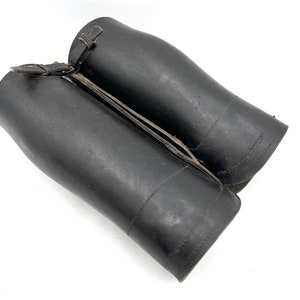The image features two black leather archery bracers, each made to be worn on the forearms. They are positioned side by side against a white background, creating a striking contrast. The bracers measure approximately six to seven inches in length and feature a belt or clasp mechanism at the top for tightening. The leather appears somewhat worn with a matte, muddy texture, indicating a lack of recent care. Each bracer has a flared design near the elbow area for mobility and comfort. Notably, there are three lines of stitching at the bottom, spaced evenly apart. Despite their utilitarian appearance, the bracers are intricately detailed, embodying both functionality and a rugged aesthetic. The light source illuminates the bracers from the top left, accentuating the stitching and the texture of the leather.